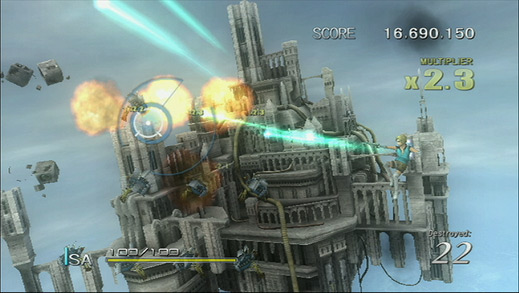A striking image of a futuristic city suspended in the sky, possibly above planets or drifting through space. The city is a marvel of architectural ingenuity, with a complex array of towers, turrets, and structures extending both above and below the main platform. On the right-hand side of the scene, an infiltrator dressed in a green jacket and dark green trousers is captured in mid-action, firing a laser weapon at various parts of the city. Their precise shots have already caused several explosions, with visible chunks of the structure being blasted away, sending fiery debris into the air. The lower edge of the image features a detailed scoreboard, prominently displaying "X-23" alongside other readings, possibly indicating magnification levels or tactical data. The background is a muted grey, providing a stark contrast to the vivid fireballs created by the laser blasts, further highlighting the intensity and chaos of the scene.